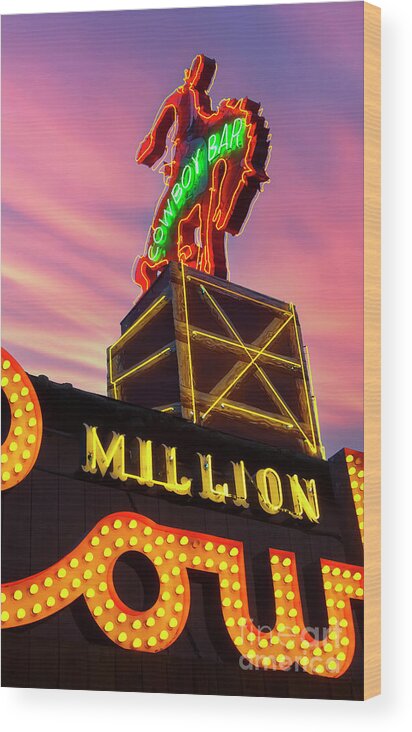The image depicts the top part of the entrance to a bar, showcasing a vibrant and detailed neon sign. At the apex of the roof, there is a large, illuminated sign featuring a man riding a rearing horse, both outlined in bright yellow neon lights. The central part of the sign highlights the words "Cowboy Bar" in green neon light. This section is set on a support structure resembling a wooden block with a lighter wooden edge and additional geometric neon patterns around it. Below the main sign, there is a rectangular box with yellow lines flanking each side, and lower down, the word "Million" is displayed in neon light. Part of the word "Cowboy" is cut off, leaving only the letters "O" and "W" visible. The background consists of a dark façade, likely the bar's exterior wall, and an enchanting sky with hues of purple, pink, and white, reminiscent of a cotton candy sunset. The overall ambiance suggests a lively and possibly Western-themed establishment.